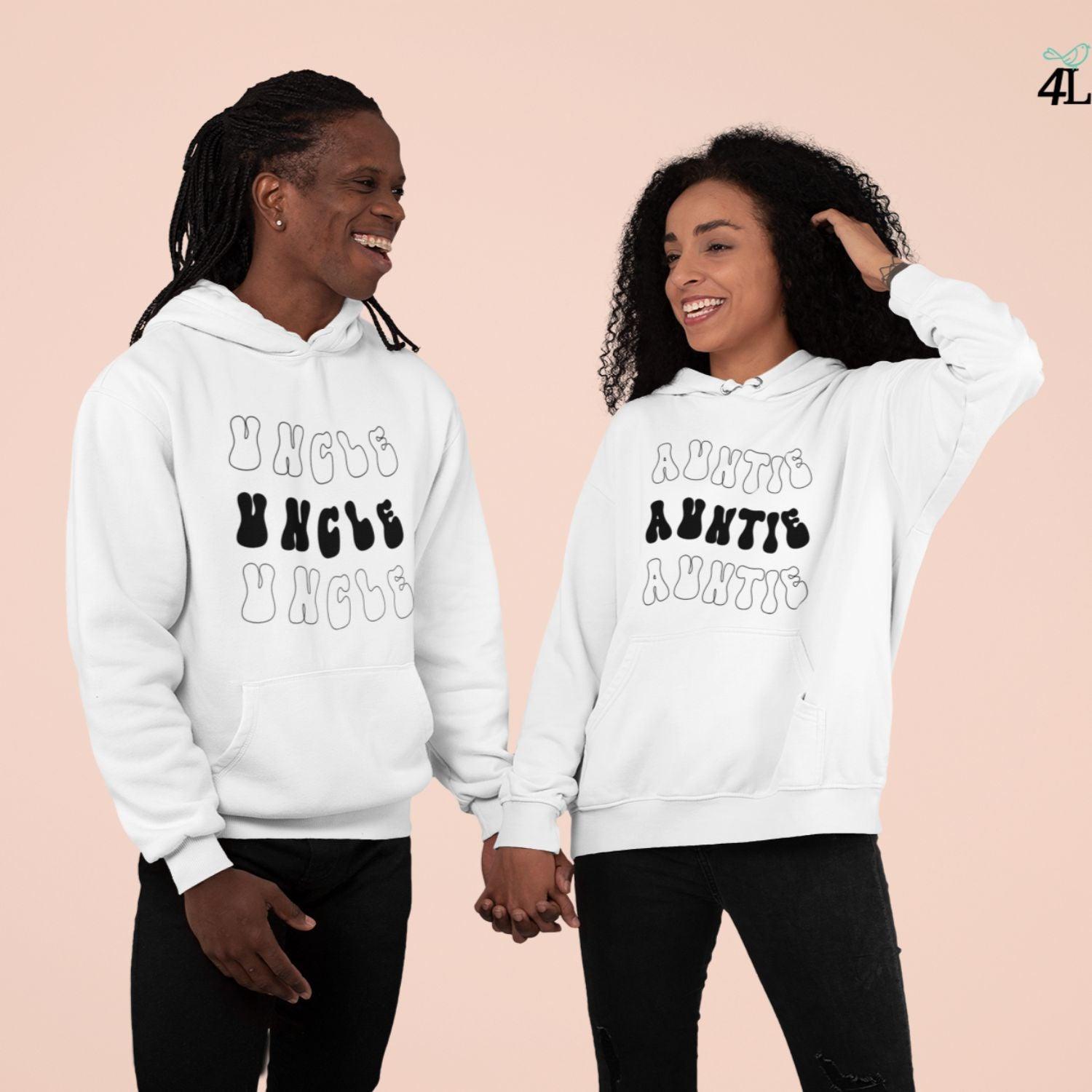In this image, a young Black couple stands hand in hand against a light peach background. Both are smiling brightly, their teeth visible. The man, standing on the left, wears a white hoodie that features the word "Uncle" printed three times: once in white with a black outline, once in solid black, and once again in white with a black outline. He has braided hair, an earring, and is dressed in black pants. The woman, on his right, wears a matching hoodie displaying the word "Auntie" in the same styles and order. She has wavy, or curly hair, and also wears black pants. Her left hand touches her hair while her right hand holds the man's. In the upper right corner of the image, a small detail shows the text "4L" alongside the image of a bird facing right.